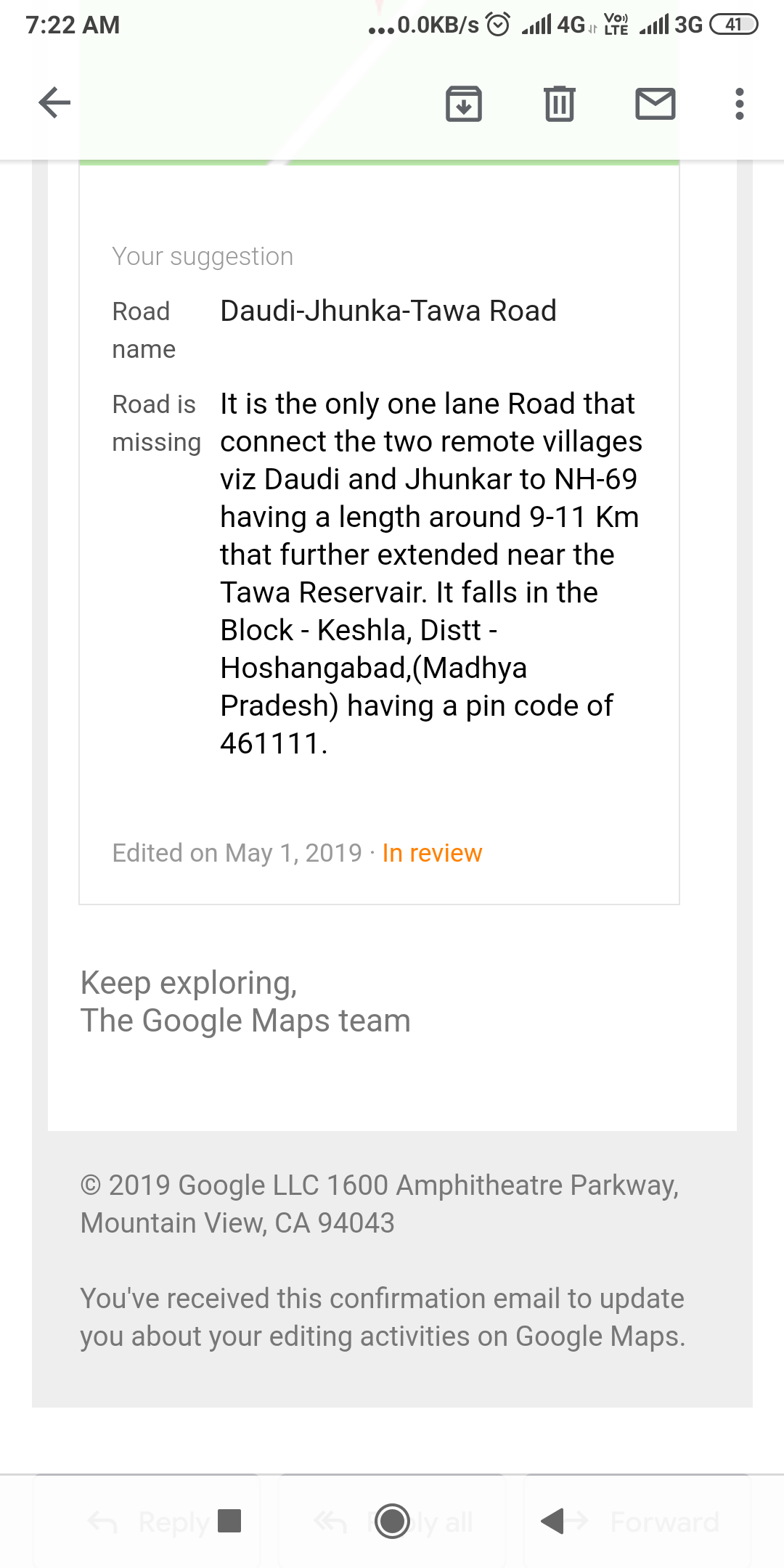This is a detailed screenshot captured from a smartphone at 7:22 a.m. The top left corner displays 0.0 kilobytes, indicating no current data usage. The phone is connected to a 4G network with full bars for both 3G and 4G signals. An alarm is also set. On the right side of the screen, the number "41" is visible, although its context is unclear.

The interface is white and features a back arrow, followed by icons for Files, Delete, Email, and a three-dot menu. A green line separates this section from the next, which contains map-related text.

The displayed text discusses a road named "Junker Tawal Road," which is incorrectly named as "Road." This one-lane road connects the villages of Via Dotti and Junkar to NH 69, extending about 9 to 11 kilometers and leading to the Toa Reservoir. It runs through the block Kashia in Hoshangabad, Madhya Pradesh, with a pin code of 461111. This information was edited on May 1st, 2019, and includes a prompt from the Google Maps team to "Keep exploring."

Below this, a gray bar states "2019 Google LLC, 1600 Amphitheater Parkway, Mountain View, California 94053." Another line explains that this email confirms updates to Google Maps editing activities, followed by playback controls and a red dot indicating recording is in progress.